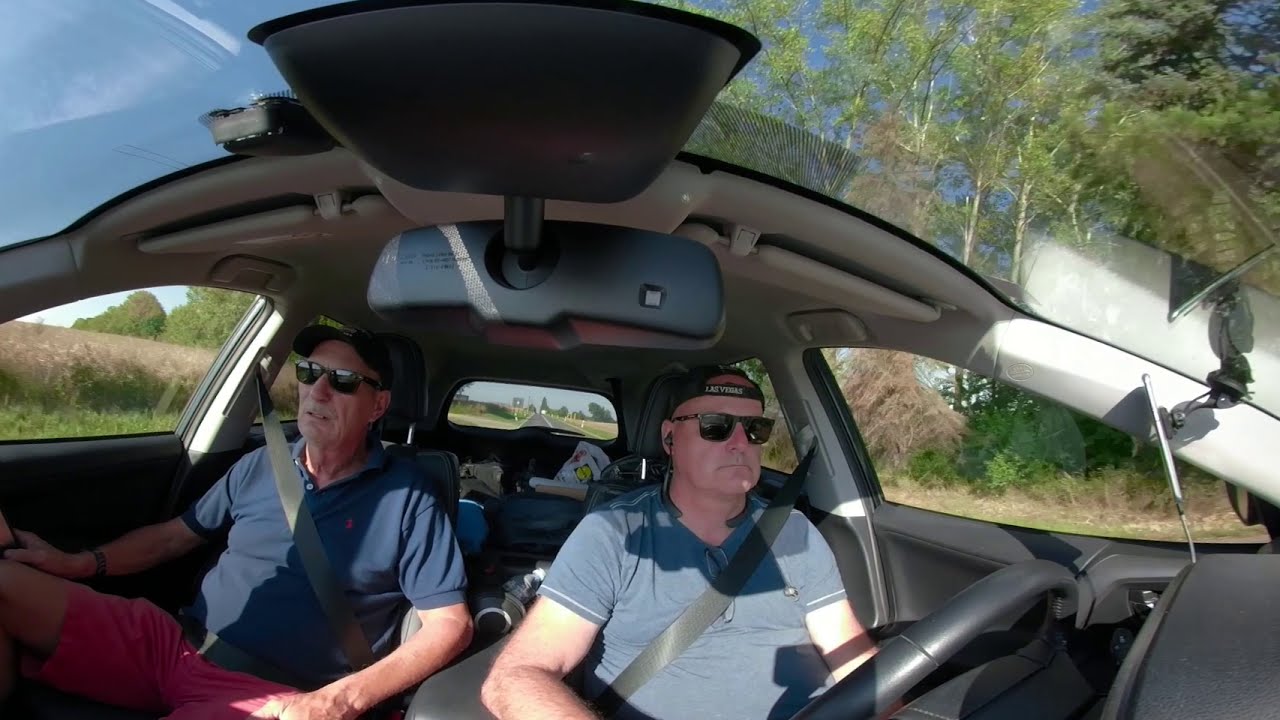In the center of the image, we see two older men seated in a car, both wearing sunglasses and ball caps. The driver, on the left, is in the front seat wearing a cap turned backward. The passenger, also in a ball cap and sunglasses, has a mustache and is dressed in a blue polo shirt with red shorts. Both men are wearing their seat belts. The image, possibly taken with a dashboard-mounted smartphone, shows a slightly distorted view capturing the inside of the vehicle. In the back seat, there are various objects, hinting at a casual, perhaps road trip setting. The environment outside the car is rural, with a grassy field and scattered trees on either side. It's the middle of the day under a bright blue sky with some clouds, adding to the vibrant colors in the scene which include black, blue, white, green, brown, orange, red, pink, and tan. The road they are on appears deserted, enhancing the serene, countryside atmosphere.